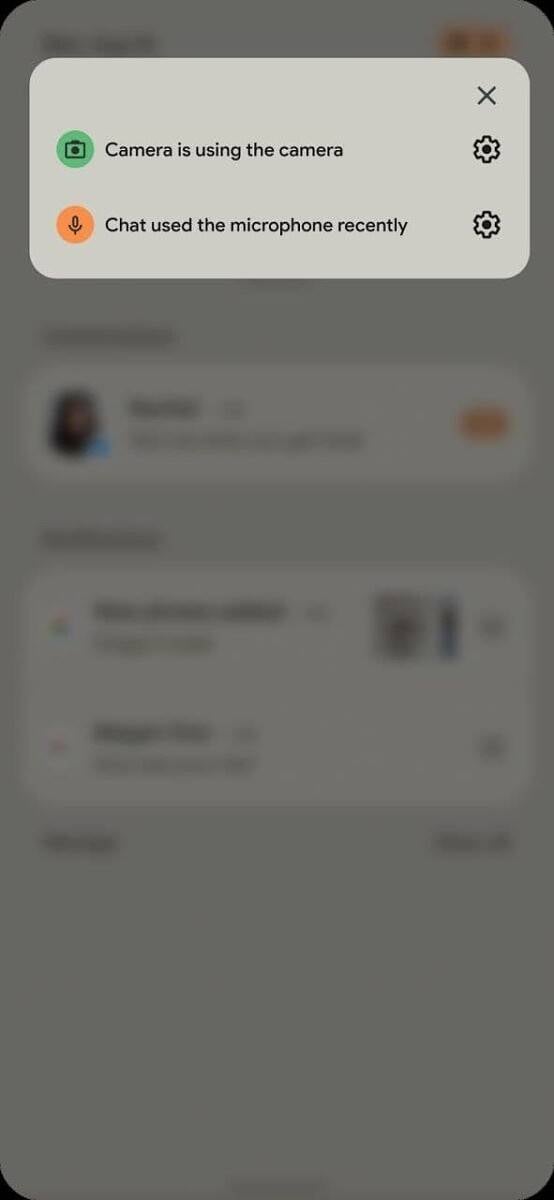A detailed screenshot is displayed, capturing a segment of a smartphone interface. At the top, various icons can be seen: a camera icon, indicating recent use of the camera, and a microphone icon, signifying recent use of voice input. These icons are distinctly colored, with the camera icon highlighted in green and the microphone icon in orange. An "X" icon is positioned for closing the window, which appears as a rounded rectangle in a gray hue. The background consists of blurred phone settings, making their details indistinguishable. The focus remains on the central notification interface, emphasizing the recent hardware usage on the device.